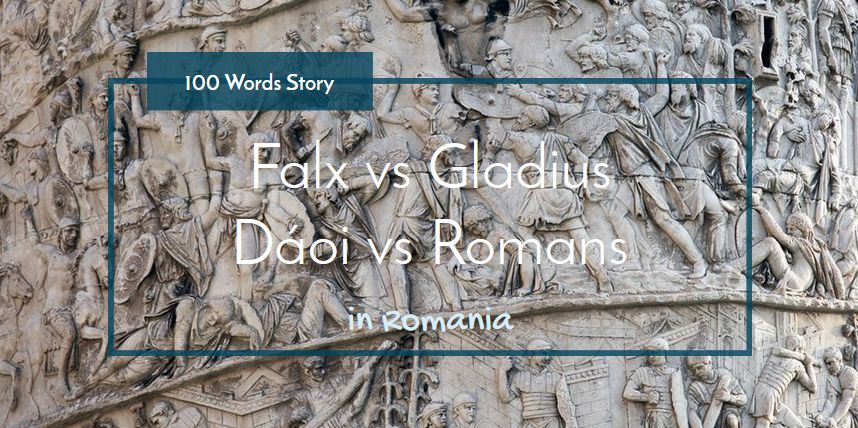This image features a highly detailed bas-relief sculpture, intricately carved and predominantly beige in color, which serves as the visual starting point for what appears to be a historical report, project, or possibly a YouTube introduction. The sculpture is divided into multiple rows, each depicting human figures in various scenes of medieval life and warfare. The bottom row shows men engaging in labor, the middle row vividly illustrates a fierce battle with soldiers wielding shields and weapons, while the top row, only partially visible, hints at additional figures.

Overlaying the center of this elaborate stone or stone-like relief is a dark blue rectangular border with white text, acting as a title or header. The text reads "A Hundred Word Story," followed by "Falks versus Gladius, Daoi versus Romans" in a bold script, and concludes with "In Romania" beneath it. The combination of the intricate sculpture and the informative text box suggests a rich historical narrative involving battles between Daoi and Romans, likely serving either as a prompt for storytelling or as a depiction of an actual historical event.